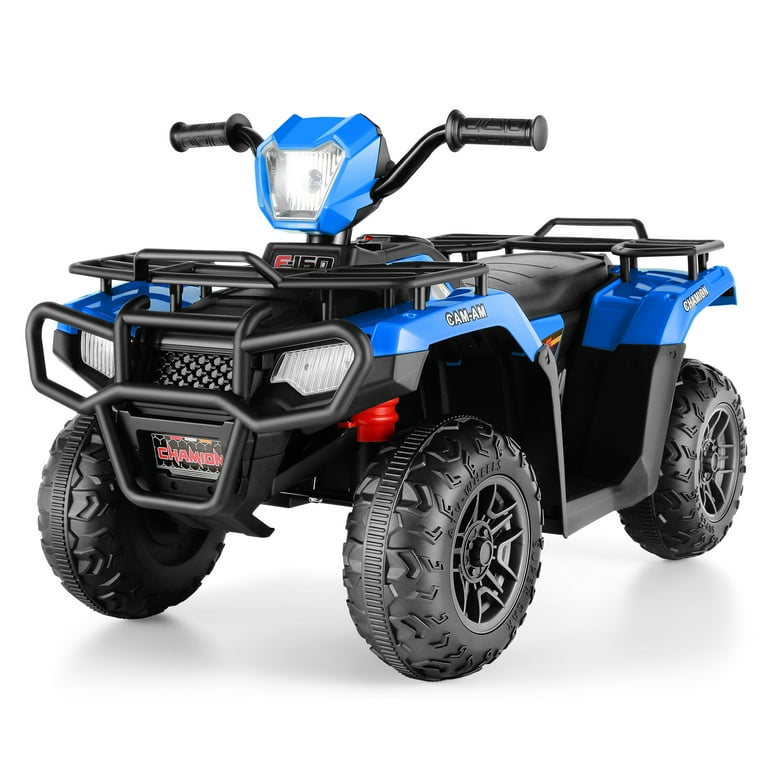The image features a sleek, shiny, and new-looking Can-Am ATV designed for off-road adventures. It has a predominantly blue body with black accents, including the handlebars and seats. The ATV boasts a distinctive design with a metal roof over the tires, also blue, and a black platform body. It has four large tires, two on each side, emphasizing its sturdy build. Notably, the front sports a "Champion" license plate and a prominent grill. The handlebars, resembling those of a motorcycle, include a headlamp with "F-150" marked underneath. The vehicle also features the lettering "Cam-Am" on the body, adding to its distinctive branding. The bright blue elements are particularly prominent on the rims or fenders, and the backdrop of the image is entirely white, further highlighting the vehicle's polished appearance.